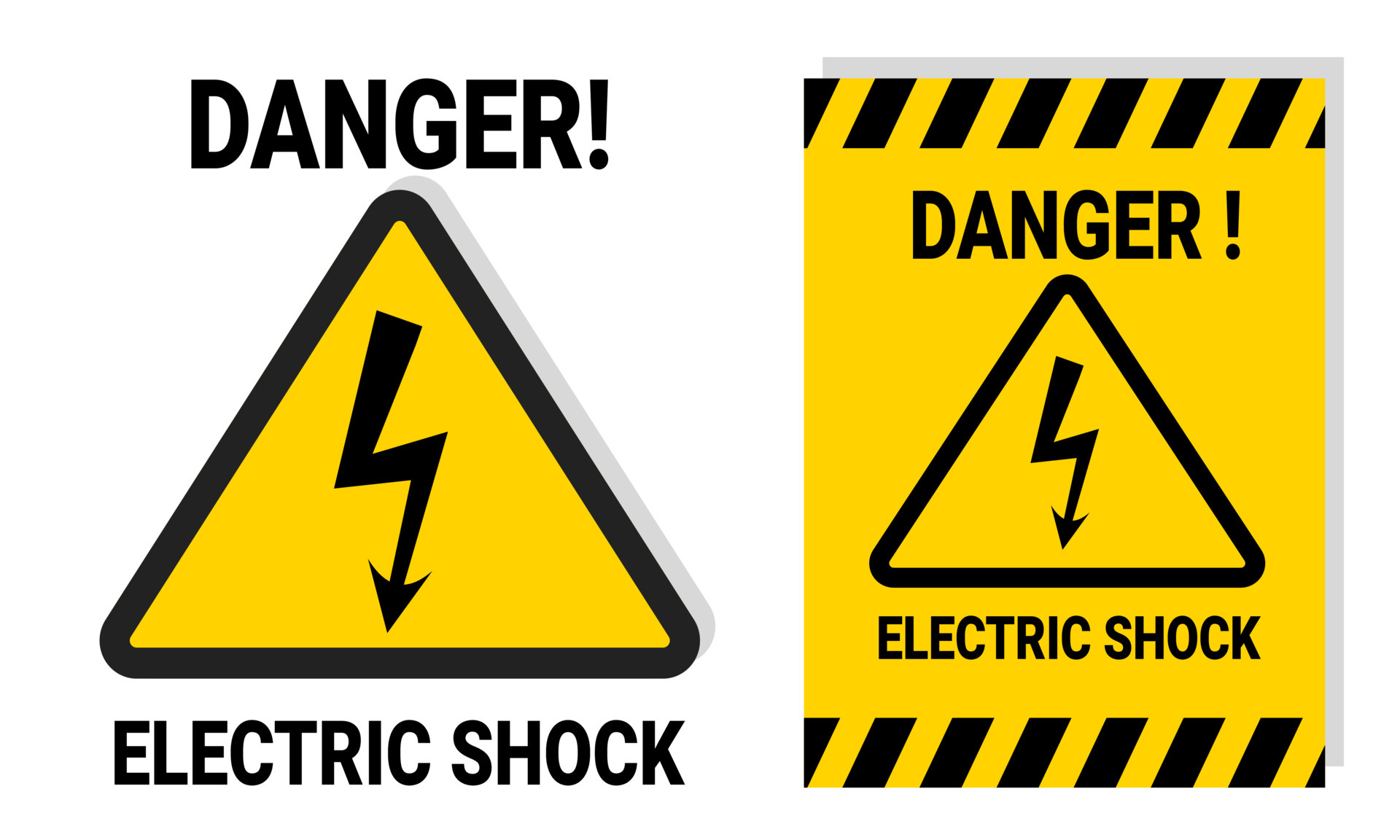The image displays two warning signs side by side, both cautioning against electric shock. On the left, the sign features a white backdrop with the word "DANGER!" written in all capital black letters above a yellow triangle bordered in black, which contains a downward-pointing black lightning bolt. Below the triangle, the words "ELECTRIC SHOCK" are also in black. The sign on the right is similar but has a yellow background with black horizontal stripes at the top and bottom edges. This sign also reads "DANGER!" in black capital letters, followed by the same yellow triangle with a black border and downward-pointing black lightning bolt. Below the triangle, the words "ELECTRIC SHOCK" appear in the same black sans-serif font. Additionally, the right sign features a light gray drop shadow, adding a subtle three-dimensional effect.